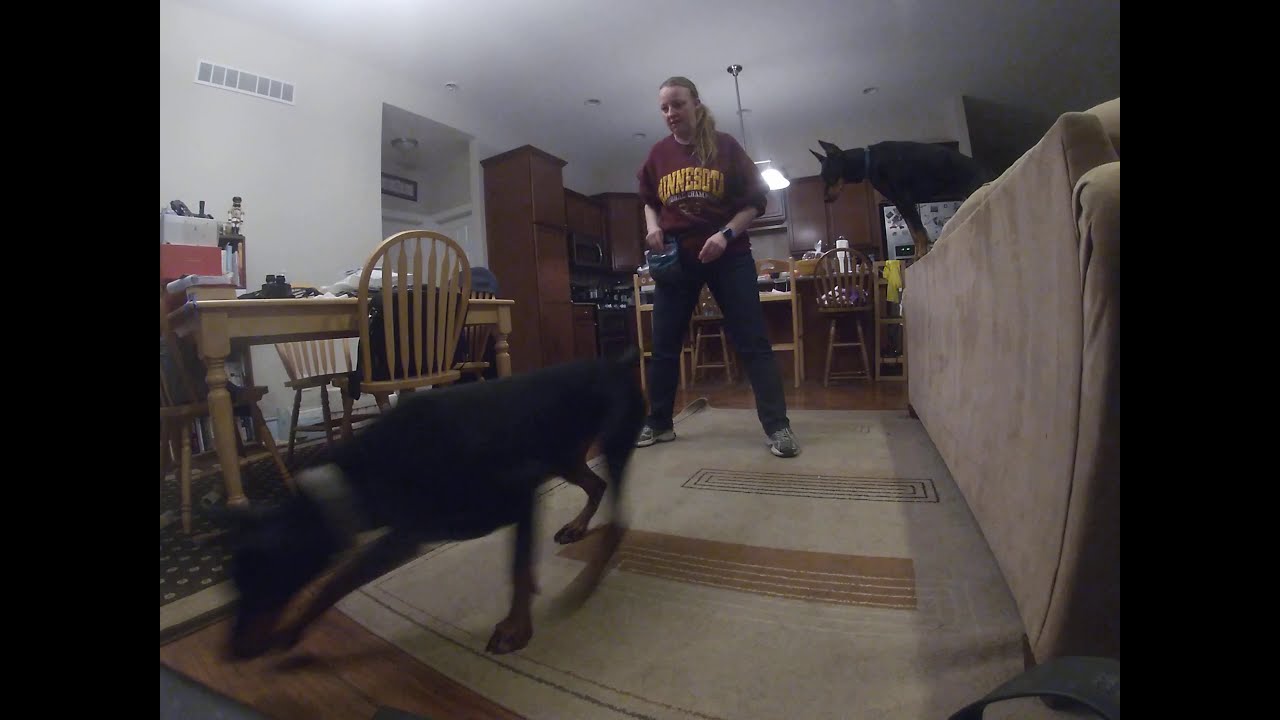The image captures a detailed indoor scene in a landscape view, framed with black borders on the right and left. At the center, a young woman with dirty blonde hair in a ponytail is wearing a dark red sweatshirt with yellow text that reads "Minnesota," black pants, a watch on her left wrist, and gray sneakers. She stands on a cream-colored rug, looking down at a mid-sized, black dog resembling a Rottweiler, which is in motion heading towards the bottom left corner of the image. In the background, on the right side, there's the back of a cream-colored sofa with another dog, also mid-sized and similar in breed, perched atop it, looking on.

The setting appears to be a well-lit kitchen, discernible by bar stools, dark brown wooden cabinets, lighting, and a white ceiling and walls. There's a wood table with four chairs to the left, cluttered with various items, possibly serving as a makeshift desk. An air vent is visible in the top left corner. In summary, the photo intricately captures the woman and her dogs in a cozy kitchen-living room area, characterized by detailed furnishings and a warm atmosphere.